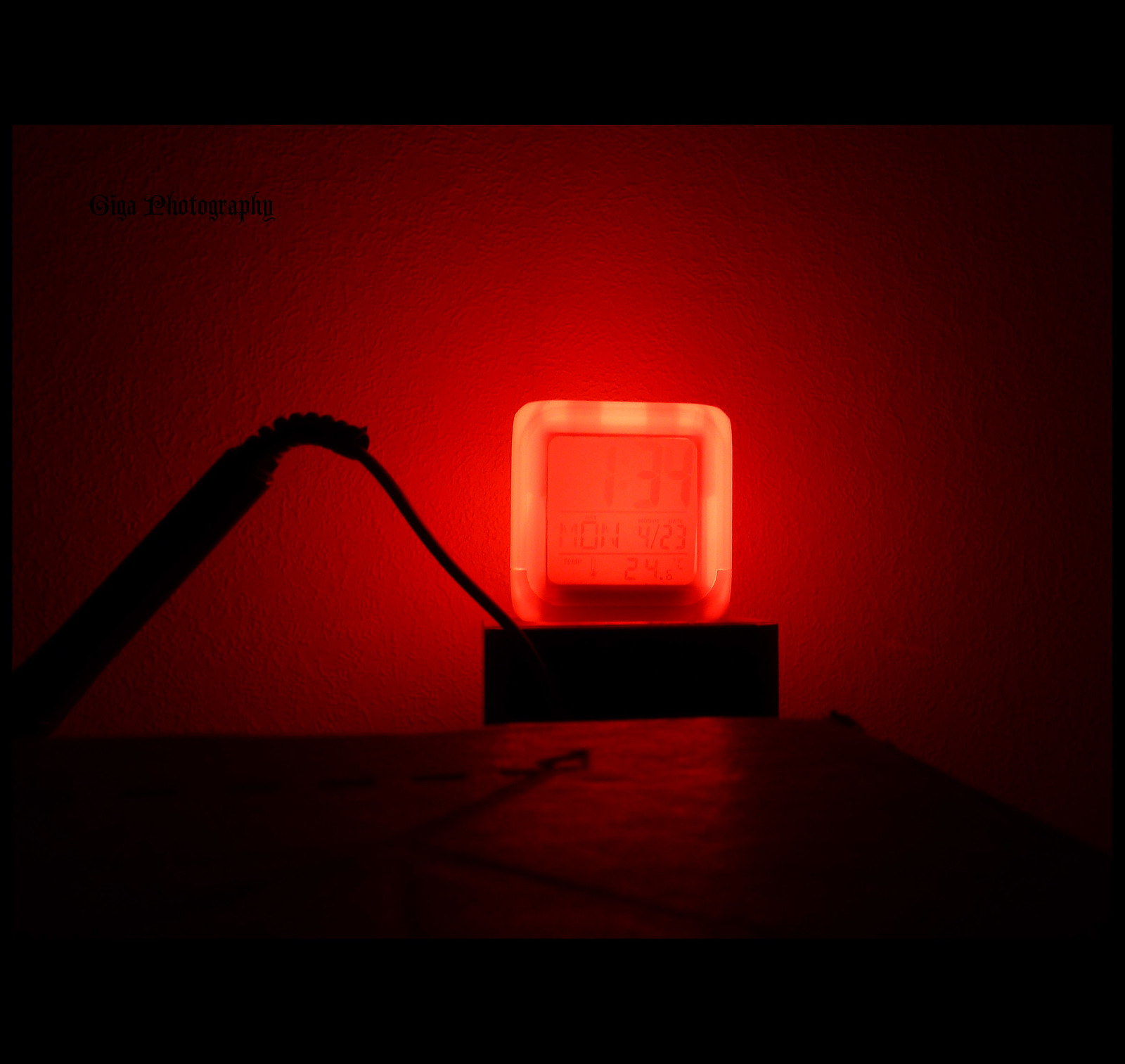The image depicts a dimly lit scene with a single light source emanating from both the top and bottom edges. At the center of the image, there is a distinct dark square, through which a vivid red light shines, possibly originating from a light source below. Surrounding the red light, a translucent or clear barrier, potentially a lens, gives the light its striking hue. Emerging from the base of this square is what appears to be a wire or a line-like object. The square itself primarily appears dark, yet features a central zone that could be darker brown over a lighter background, such as beige, white, or transparent, colored by the red light. The background wall is lightly colored, catching the reflection of the red glow. At the bottom foreground of the image, there is a flat, dark surface, contrasting with the illuminated elements above it.